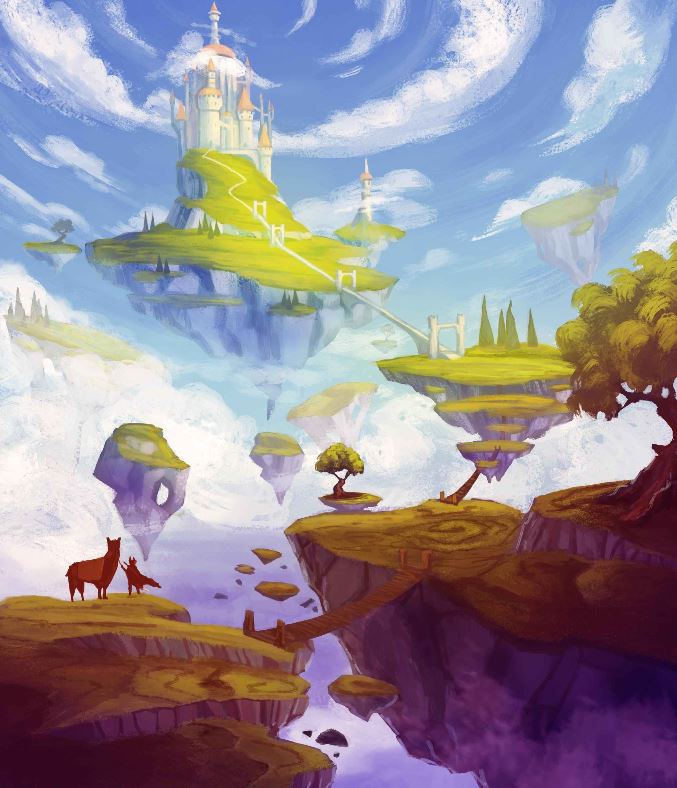This detailed digital artwork, which resembles a cartoon or video game scene, features a fantastical landscape of floating islands connected by various bridges. Each floating island appears distinct with vibrant greens, browns, and yellows set against a bright blue sky dotted with white, fluffy clouds.

At the topmost level, a majestic white and tan castle with orange and purple accents stands proudly on an island. This island is connected by a white stone bridge to a second, smaller island marked by a green meadow and a prominent, white stone archway.

Descending further, a third island, darker and rocky with a gnarly old tree, links to the second via a dark wooden bridge. Another bridge extends from this island to a fourth, where a variety of animals can be seen, including what looks like a llama and possibly a wolf or another reddish-brown creature. 

In the lower left-hand corner, a bridge leads to yet another floating island. Surrounding these islands are several smaller, mini-islands sporadically placed, enhancing the dreamy, fantasy atmosphere. 

The scene is crowned by swirling white clouds on this bright, windswept day, adding to the magical, suspended nature of this floating world. Some distant islands feature simple landscapes with single trees or additional structures, emphasizing the intricate and whimsical nature of this imaginative setting.